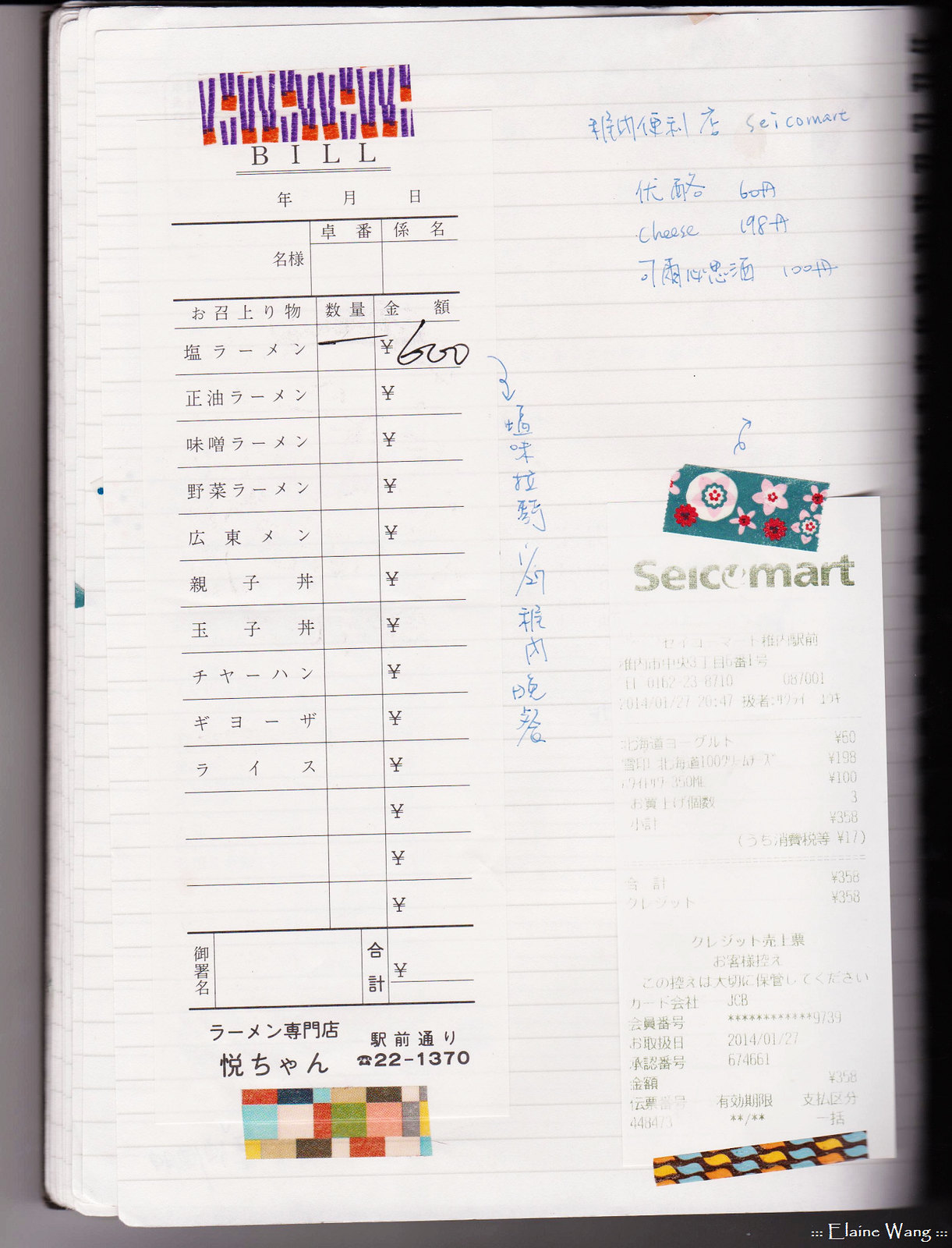In this rectangular photo, we see an open notebook with spiral binding along the right vertical edge. The notebook's white, lined pages have the word "Bill" written in the upper left corner. Below "Bill," there are three columns of Asian writing. Adjacent to these columns, on the right side of the notebook page, there is a small rectangular piece of tape adorned with floral patterns in white, red, and blue. This tape secures a faded white receipt onto the notebook. The receipt's heading reads "Psycho Mart," but the rest of the text is in an Asian alphabet, making it unreadable.